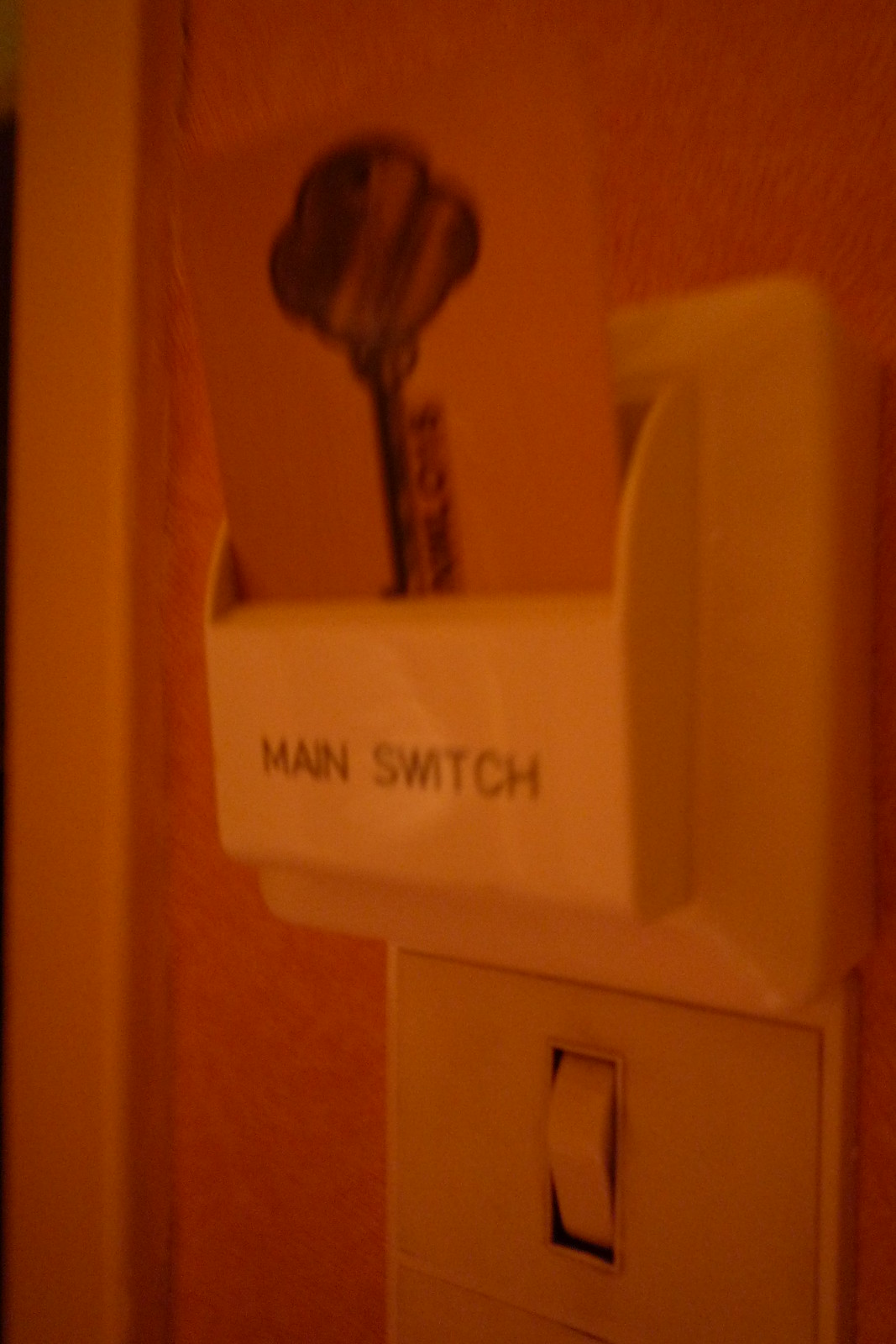The image portrays a close-up of a wall painted in a dimly lit coral color, which casts a warm and somewhat shadowy ambiance over the scene. On the left side of the frame, there is a door frame, likely white or off-white, though the dim lighting makes it difficult to discern its exact shade.

Prominently featured in the lower right-hand side of the image is a white plastic light switch with an off-white rectangular panel. The switch is in the down position, nestled within a rectangular wall plate. Above this switch is a small, white compartment that resembles a mini mailbox or shelf. The compartment has an inscription in black letters that reads "MAIN SWITCH."

Inserted into this compartment is an orange card, which harmonizes with the coral hue of the wall. The card showcases an illustrated image of a black, old-fashioned key. The key is oriented vertically, pointing downward. Its design includes a top portion vaguely reminiscent of a three-leaf clover, augmented with dark streaks and edges that give it a burnt, rustic appearance.